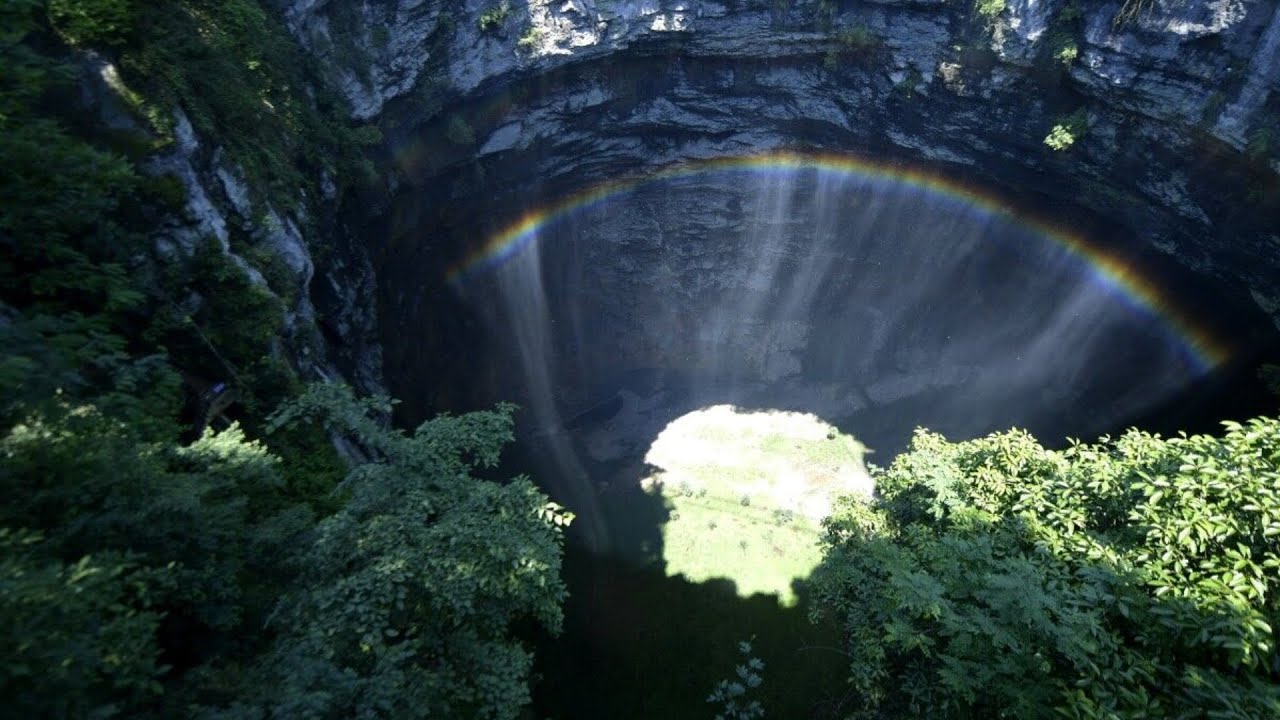This captivating outdoor photograph, likely taken from an elevated vantage point such as a cliffside or from a drone, offers a mesmerizing view down into a ravine or canyon area framed by lush, dark green foliage. The dense, vibrant green trees on either side have thick leaves, obscuring the branches entirely. At the bottom, the ground appears a dark light green with patches of yellow dirt. High above, the rocky ceiling of the canyon, composed of light gray and light blue stones, creates a shadowy arch overhead.

Prominent in the image is a striking rainbow, which stretches across the top of the arch in hues of blue, yellow, and orange, casting a soft white light down through the opening. On either side of the canyon walls, green vegetation intertwines with white rock, adding to the scene's earthy palette. There are also some white flowers towards the center and an interplay of shadows and light creates a dynamic contrast, with sunlight streaming through to illuminate the middle of the clearing, producing the radiant rainbow effect.

In the background, the rocky wall is visible, adding to the sense of depth and scale in the image. No people or text are present, allowing the natural beauty and serene atmosphere of the scene to speak for itself. The view encapsulates the tranquility and rugged beauty of a canyon enveloped in diverse and vibrant natural elements.